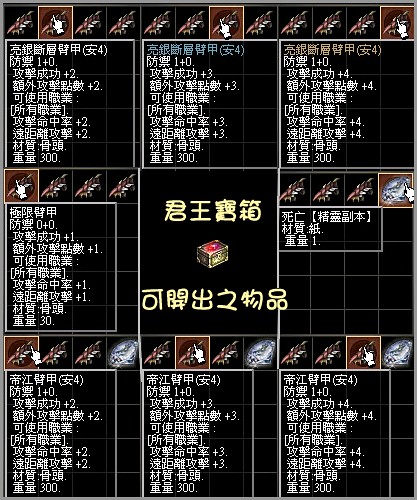The image showcases a digital display predominantly featuring Chinese text on a black background, overlaid with a thin gray grid pattern. The centerpiece is a yellow and bronze treasure chest with a latch, slightly tilted to the right. Atop this chest sits a glowing red gem. Around this central image are stylized Chinese characters, occasionally giving the impression of Korean due to their circular design. The display includes repeated elements such as video game-like assets: diagonal red and gray spikes, diamond-like jewels tilted slightly leftward, and ashlar-cut gems. Several white cursor hands hover over various items, highlighting the associated Chinese text. These cursors indicate different interactive elements or buttons, with sections of text appearing at the top, bottom, left, and right of the display. Additionally, there are numerical elements embedded within the text, like sequences of "1+0," "1,3," and the number "300." The overall aesthetic is that of an oriental chart or interface, rich in foreign language details and gaming iconography, with nothing presented in English.